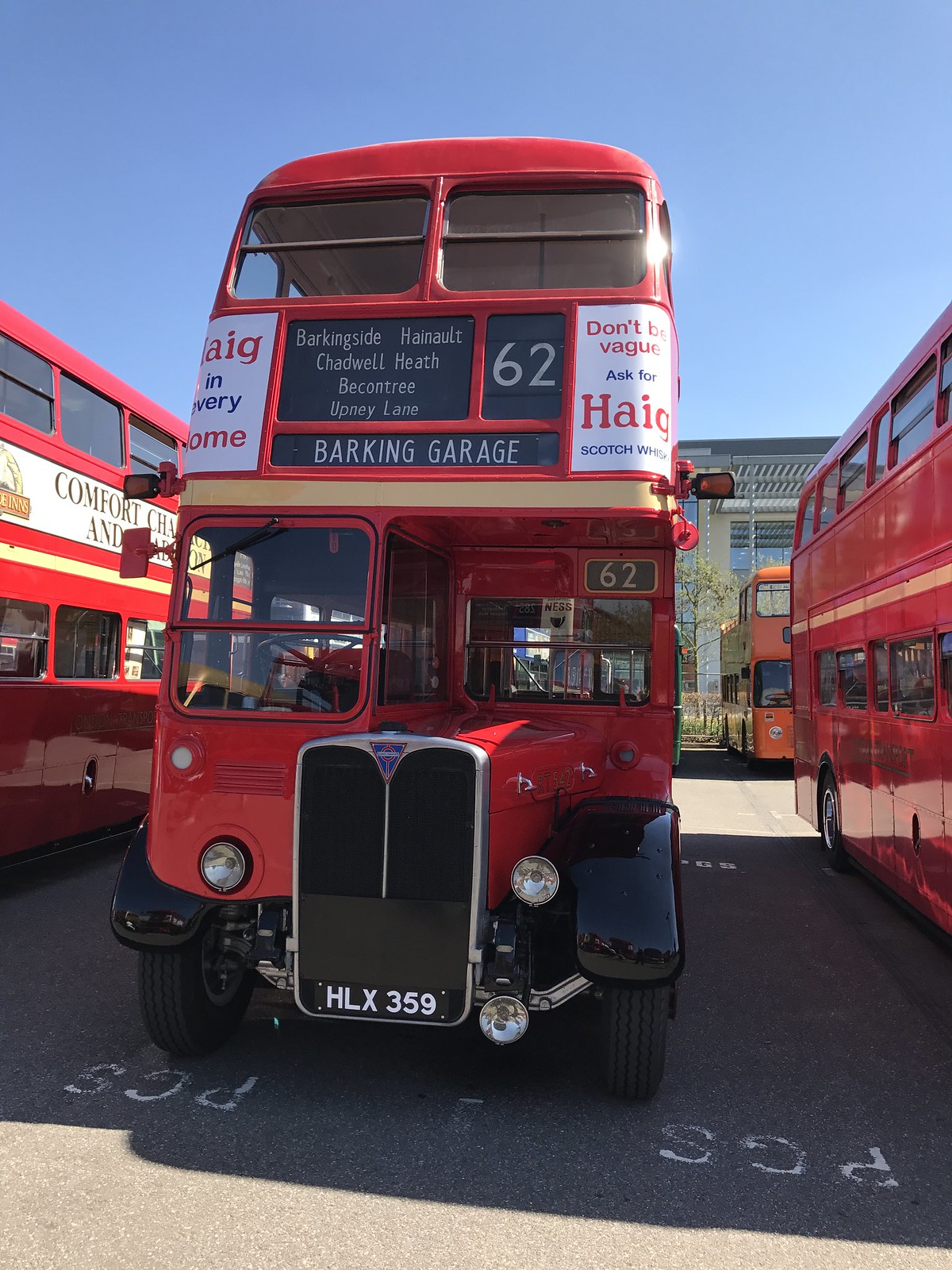This is a detailed color photograph of a classic London-style double-decker bus parked on an asphalt lot, surrounded by several other identical red buses. The focus is on an antique, bright red bus with black fenders and trim. The bus, distinguished by its rectangular black grille and license plate numbered HLX-359, is centered in the image, occupying a marked parking space. Above the grille are its distinctive double windshields, and at the very top, a black destination sign reads "Barking Garage," with service details including "Barkingside, Hainault, Chadwell Heath, Becontree, Upney Lane." The bus is numbered 62, prominently displayed at both the lower and upper sections. Flanking the destination sign are white advertisements with red and black text; the visible ad on the upper left corner reads, “Don’t be vague, ask for Haig,” likely referencing Haig whisky. The backdrop features an office building with a white wall and a window, under a clear blue sky. Additional red double-decker buses are aligned on both sides and in the background, indicating this area serves as a parking spot for these iconic vehicles.